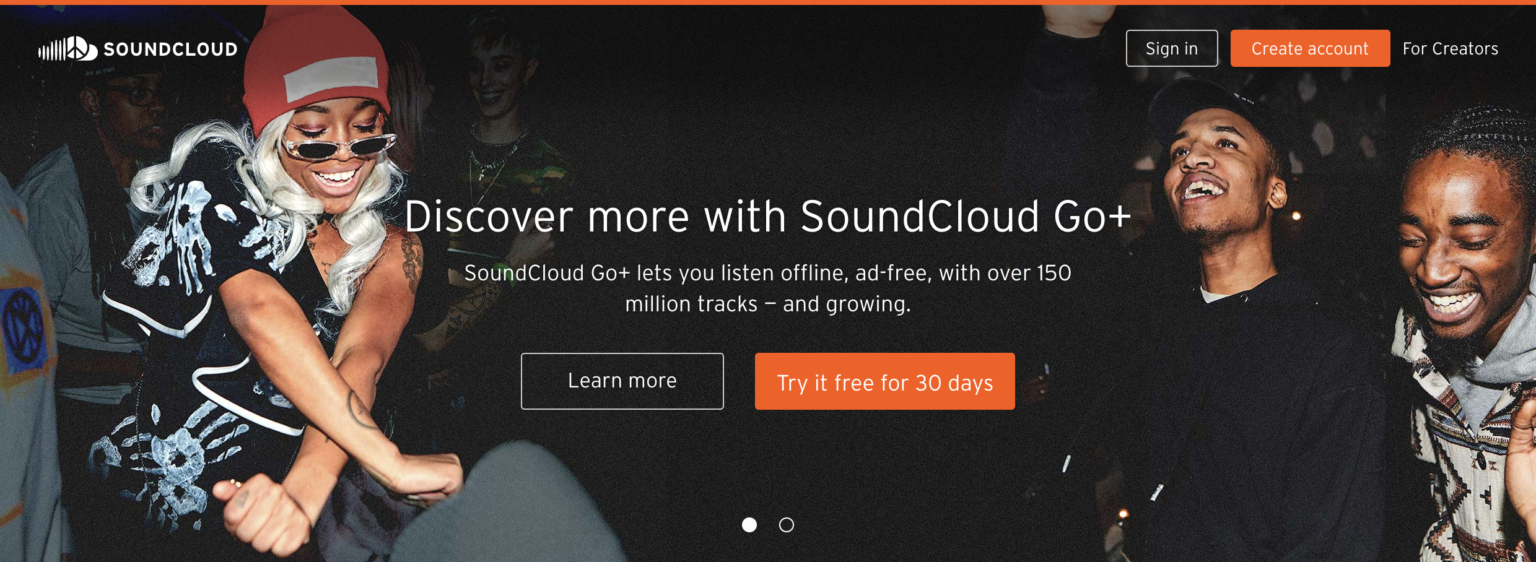Cropped screenshot of the SoundCloud website's header with a dynamic party scene background featuring people dancing. At the top left, there's an overlay with the SoundCloud icon. The center of the image prominently displays a promotional banner that reads, "Discover more with SoundCloud Go Plus." Below this, additional text explains, "SoundCloud Go lets you listen online ad-free with over 150 million tracks and growing." On the bottom left, there's a 'Learn More' button, while to its right, a call-to-action states, "Try it here for 30 days" beside an orange button. In the top right corner, a small box prompts users to 'Sign In,' with adjacent options to 'Create an Account' and a 'For Creators' link in smaller white font. Two navigation dots at the bottom center indicate that this is the first of multiple images, with the first dot colored white and the second dot black.